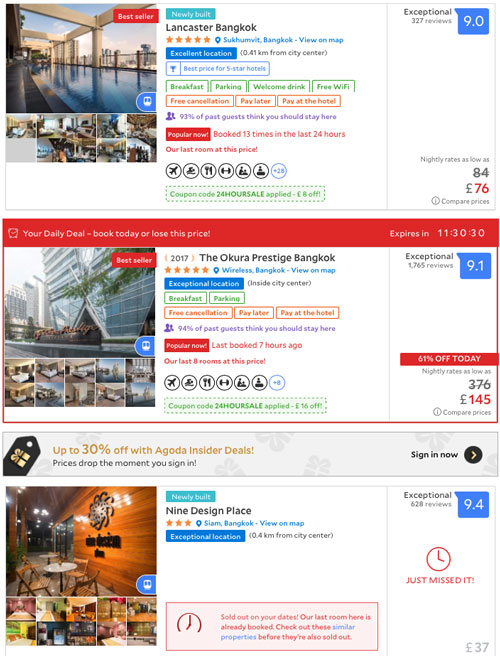The image is a vertically oriented travel website page showcasing three different places to stay, each presented in a horizontal box.

At the top is Lancaster Bangkok, featuring images and photos of the destination. This accommodation boasts an excellent location, rated 9.0. Nightly rates are shown, with an initial price of £84 crossed out and a discounted rate of £76 displayed underneath.

The second destination, highlighted in a red box with a red strip at the top, is Okura Prestige Bangkok. Accompanied by travel and destination photos to the left, this exceptional location offers amenities such as breakfast, parking, free cancellation, and options for payment both later and at the hotel. Rated 9.1 and deemed exceptional, it is currently available at a 61% discount, priced at £145 down from £376. A countdown timer indicates that this daily deal expires in 11:30:30, urging users to book immediately to secure the price.

The final listing is for 9 Design Place, featuring photographs of the resort. Rated an exceptional 9.4, it is unfortunately sold out for the user's selected dates, with a message stating, "Just missed it! Our last room here is already booked."

Between the second and third advertisements, a thin strip promotes up to 30% off with Agoda insider deals, encouraging users to sign in.

The website's color scheme includes white, blue, green, red, and pastel colors for the photographs, contributing to an inviting and visually appealing design.